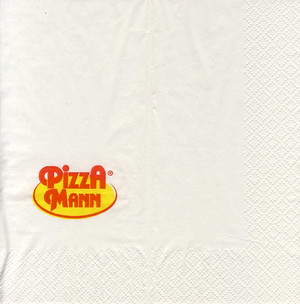The image is a close-up photograph of a white, fabric-like square napkin featuring a distinctive logo in its lower right corner. The primary material has a linen texture, and along the bottom and right edge, there is a pattern of small, perforated diamonds. The logo consists of the words "Pizza Man," with "Man" uniquely spelled with two Ns. The text is in red and is set against a yellow oval background with a red border. Notably, the A in "Pizza" is capitalized, as are the P and A, making them larger than the other letters. The overall design is traditional and simple, focusing on the fabric's minimalistic aesthetic and the brightly colored logo.